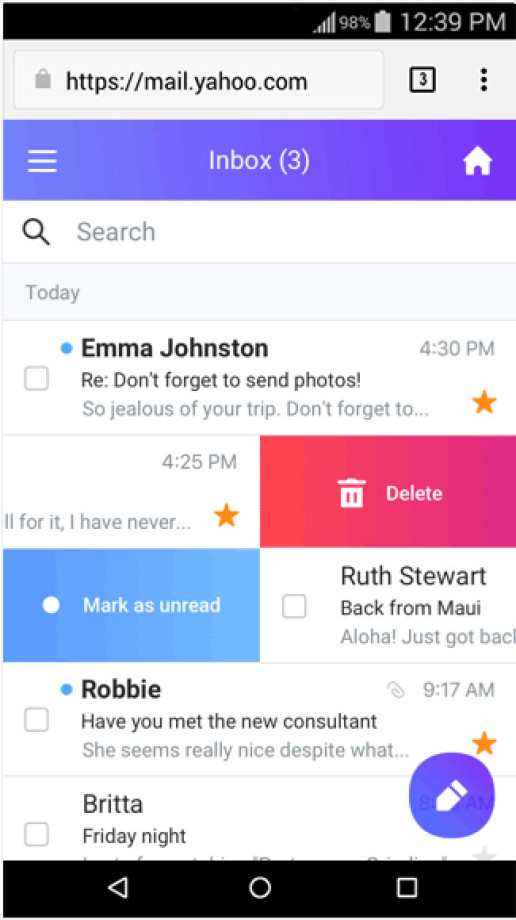This image is a screenshot taken on an old Android device, evident from the dated design of the status bar. The device shows full cell reception, a battery level at 98%, and the time is 12:39 p.m. The screenshot captures the Yahoo Mail inbox opened in a web browser, not an app, as indicated by the presence of the address bar displaying "mail.yahoo.com" and showing three open tabs.

Below the address bar, a blue banner indicates the mailbox section. It features a hamburger menu on the left, the label "Inbox," and a home button. Situated right below the banner is a search box for emails.

The main portion of the screenshot displays the list of emails. The top email is from Emma Johnston with the subject "Don't forget to send photos," received at 4:30 p.m. The second email appears in the process of being deleted, with the delete option selected but not yet confirmed. The third email is marked for being set as unread, although this action has not yet been completed.